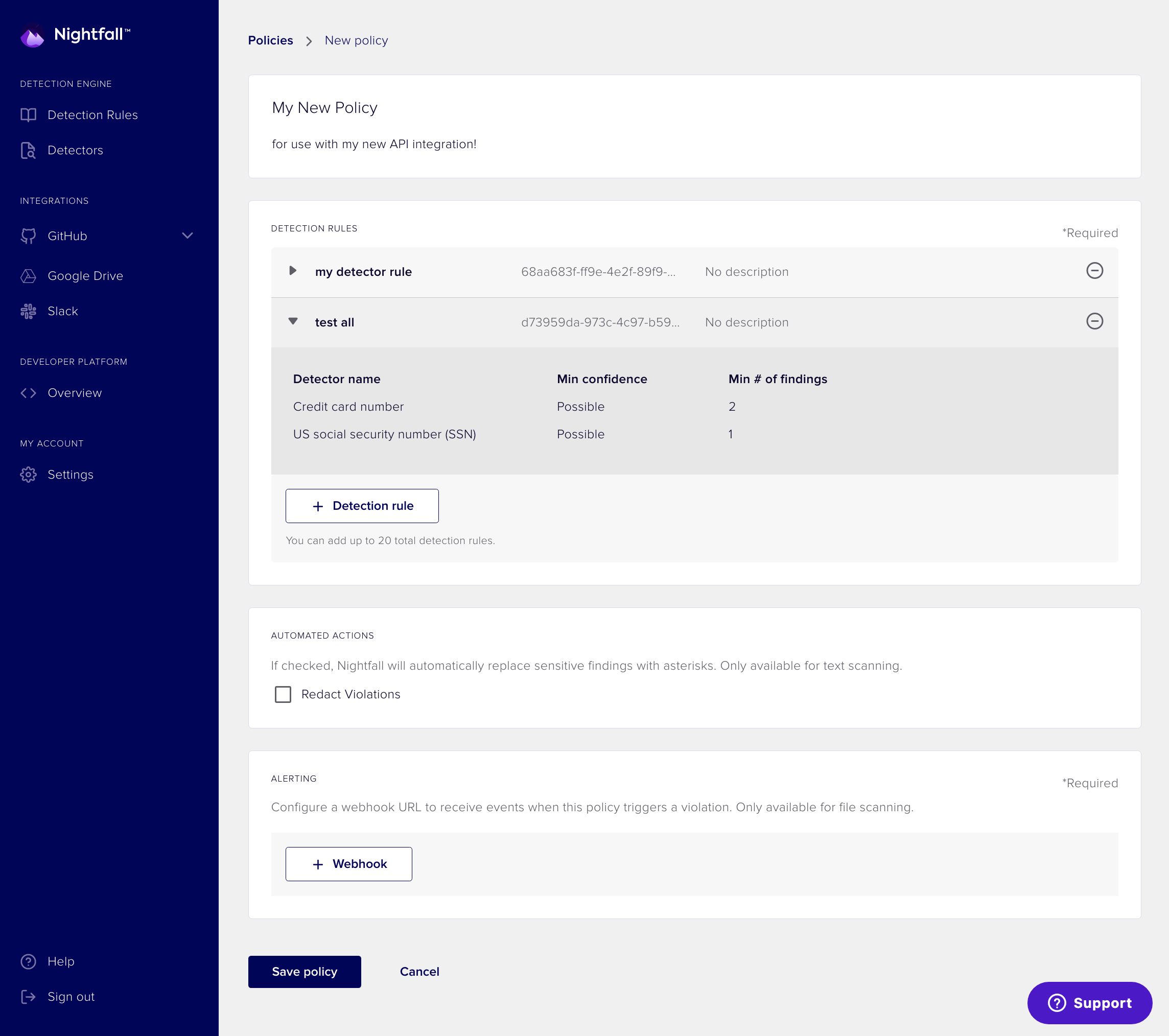Screenshot of the Nightfall Dashboard:

The image captures the interface of a platform called Nightfall. Prominently displayed at the top is the Nightfall logo, resembling a lavender tulip. The interface's primary color scheme features blue for critical elements against a gray background.

**Top Navigation**:
- Detection Engine
- Integrations
- Developer Platform
- My Account

**Main Section**:
- Policies
  - New Policy: Displays the interface for creating a new policy.

**Policy Configuration**:
1. **Policy Name**:
   - `my new policy` (within a white text box, for use with API integration)

2. **Detection Rules** (heading):
   - An asterisk (*) indicates fields are required.
   - Example: `my detector rule` without a description, and a test feature (`test all`) that also lacks a description.

3. **Detector Settings**:
   - **Credit Card Detector**:
     - `Detector Name`
     - `Minimum Confidence`: Set to `possible` because 2 findings were detected, indicating potential exposure of a credit card number.
   - **U.S. Social Security Number Detector**:
     - `Minimum Confidence`: Also set to `possible` due to 1 finding.
    
4. **Add Detection Rule**:
   - An additional field to input up to 20 total detection rules via a white box labeled `+ detection rule`.

5. **Automated Actions**:
   - **Redact Violations**:
     - A feature (toggled with checkboxes) that automatically replaces sensitive data with asterisks (applicable only for text scanning).

6. **Alerting**:
   - Another white box tagged with `*required`:
     - Configures a webhook URL to receive notifications when the policy is violated (available only for file scanning).
     - A blue box with a plus sign labeled `+ web hook` is present for adding this URL.

**Bottom Actions**:
- **Save Policy** (blue box)
- **Cancel** (blue text link)
- **Support** (blue box)

Each section is organized in a clear and concise manner, allowing users to efficiently configure and manage their data protection policies.